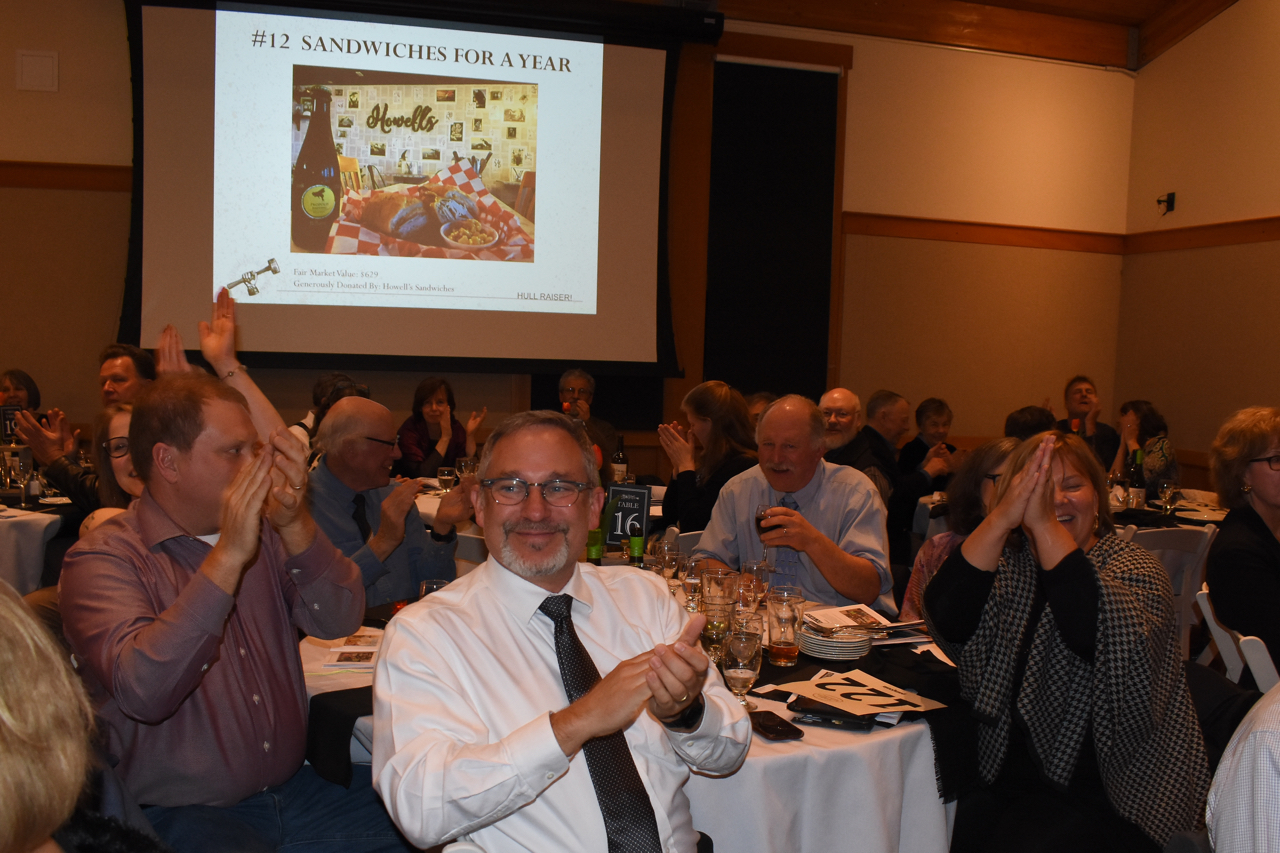The photograph captures a lively auction banquet, likely for charity, held in what appears to be a dimly lit conference room with a mixed white and gray color scheme. Numerous round tables draped in white tablecloths are filled with elegantly dressed attendees, all seated and clapping enthusiastically. Central to the scene is a man in a white button-up shirt and black tie, wearing spectacles, who joins in the applause. In the background, a large projector screen displays the text "Number 12: Sandwiches for a Year," along with an image of a sandwich, accentuating one of the auction items. The screen has a white backdrop, matching the overall decor. Scattered on the tables are papers with printed numbers, indicative of the auction process, with one sign reading "122," adding to the sense that bids have just been placed.